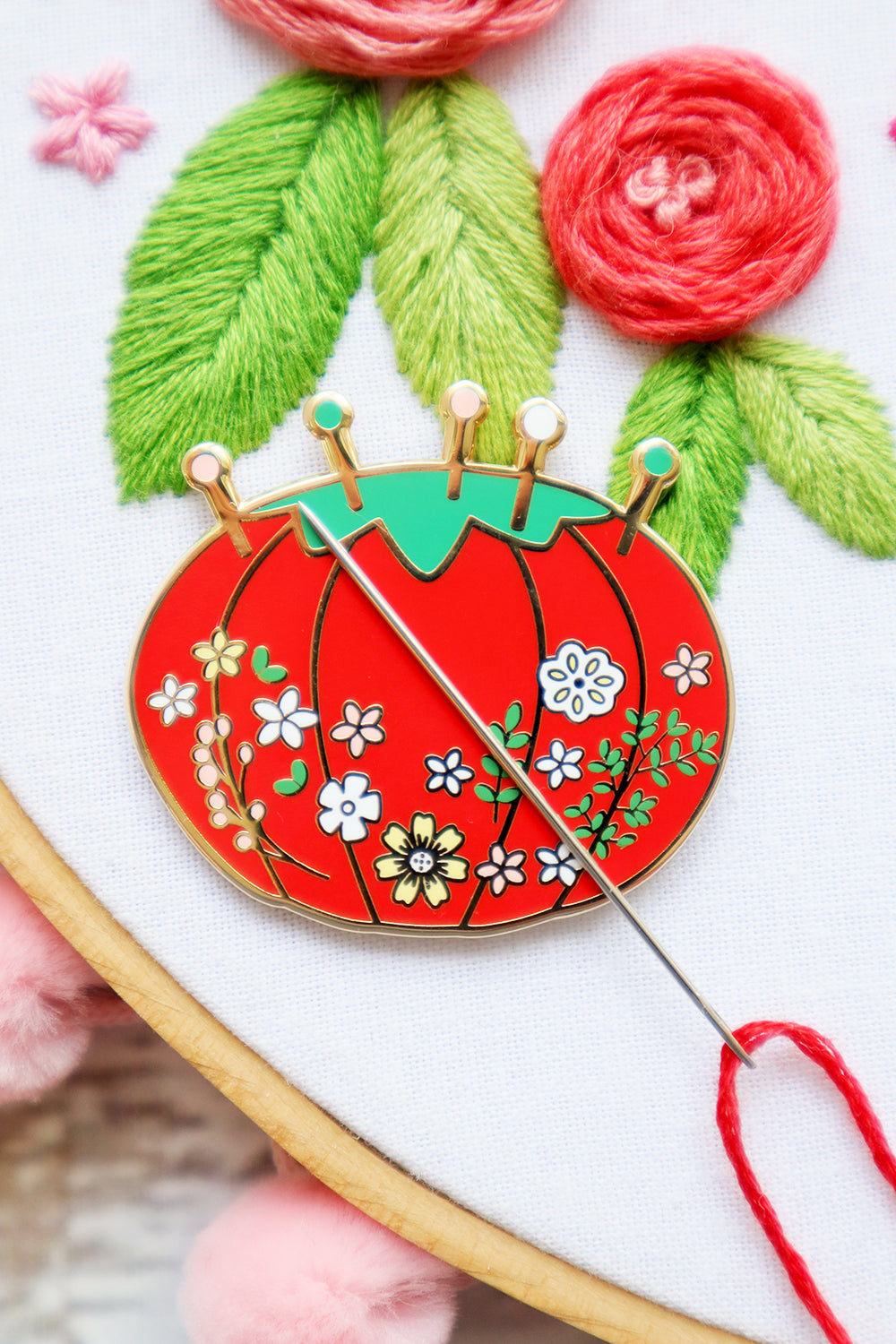The image depicts a round wooden embroidery hoop holding a white fabric backdrop, stretched taut for needlepoint. On the fabric, two large red roses are meticulously embroidered, each adorned with two green leaves. Close to these roses, a smaller pink cross-stitched flower adds a delicate touch. In the foreground, a threaded needle with red thread rests, poised for the next stitch. Additionally, there is a ceramic medallion resembling a tomato pincushion, replete with a bronze outline, a green top, and several multi-colored flowers surrounding its base. Five pins protrude from the top of the tomato, enhancing the detailed setting. Beneath the embroidery hoop, a pink cloth provides a subtle background contrast, completing this quaint sewing scene.